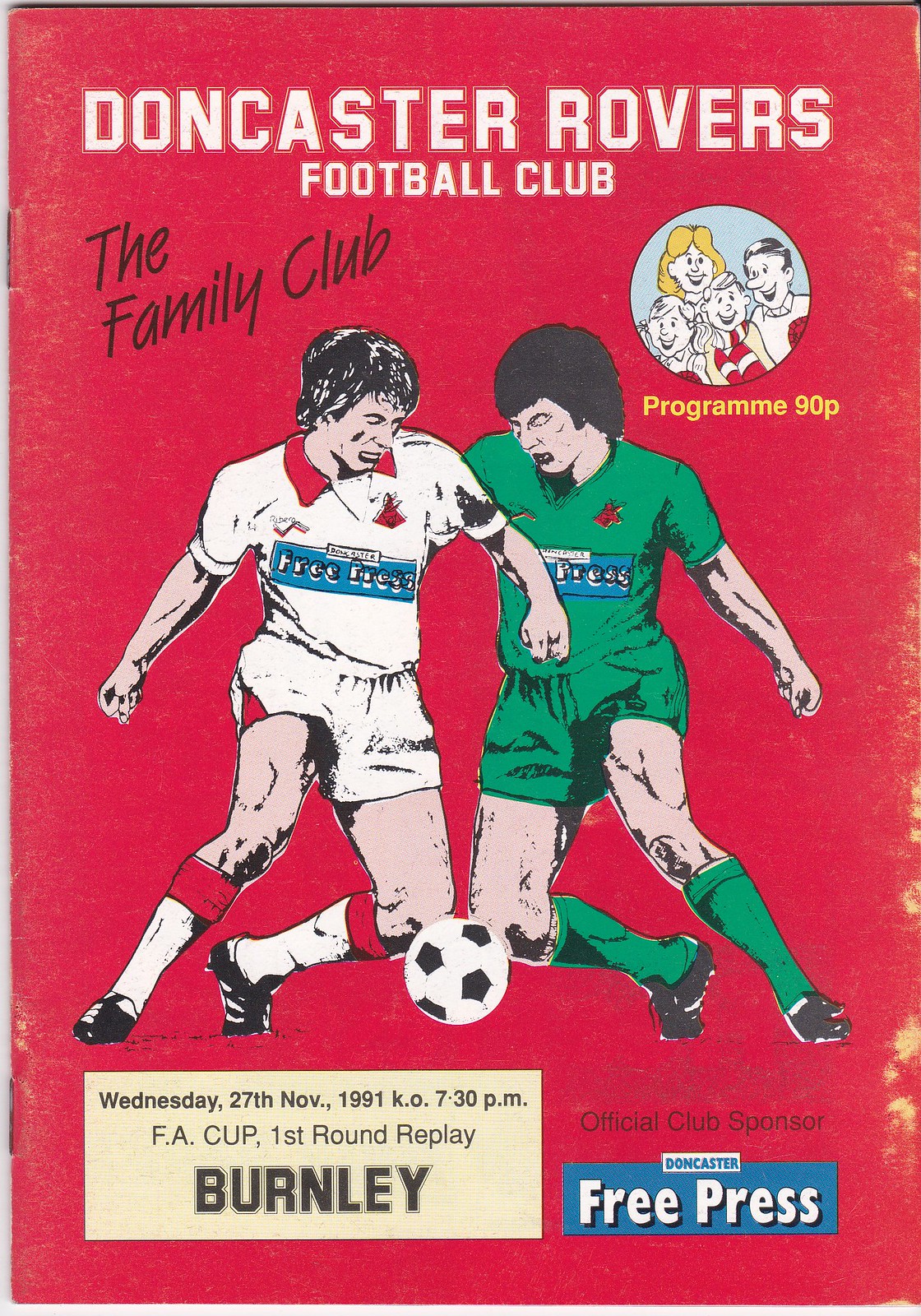This image is a vintage football club program cover in portrait orientation, featuring a bold red background. At the top, white lettering announces “Doncaster Rovers Football Club,” with “The Family Club” written in black diagonally on the left. A small circle on the right contains an illustration of a smiling family, emphasizing the club's community focus. Below, two soccer players are depicted in mid-action with a black and white soccer ball at their feet. The player on the left is dressed in a white jersey with a red collar, while the player to the right wears a green jersey and green socks. Both jerseys display the Doncaster Free Press logo on the chest. At the bottom left, a cream-colored text box details the event: “Wednesday, 27th of November, 1991, KO, 7.30 p.m. FA Cup First Round Replay, Burnley.” Additional text indicating "Program 90P" and the sponsorship by the Doncaster Free Press is also included. The cover’s aged and slightly worn appearance, complete with visible staples, adds to its nostalgic charm.